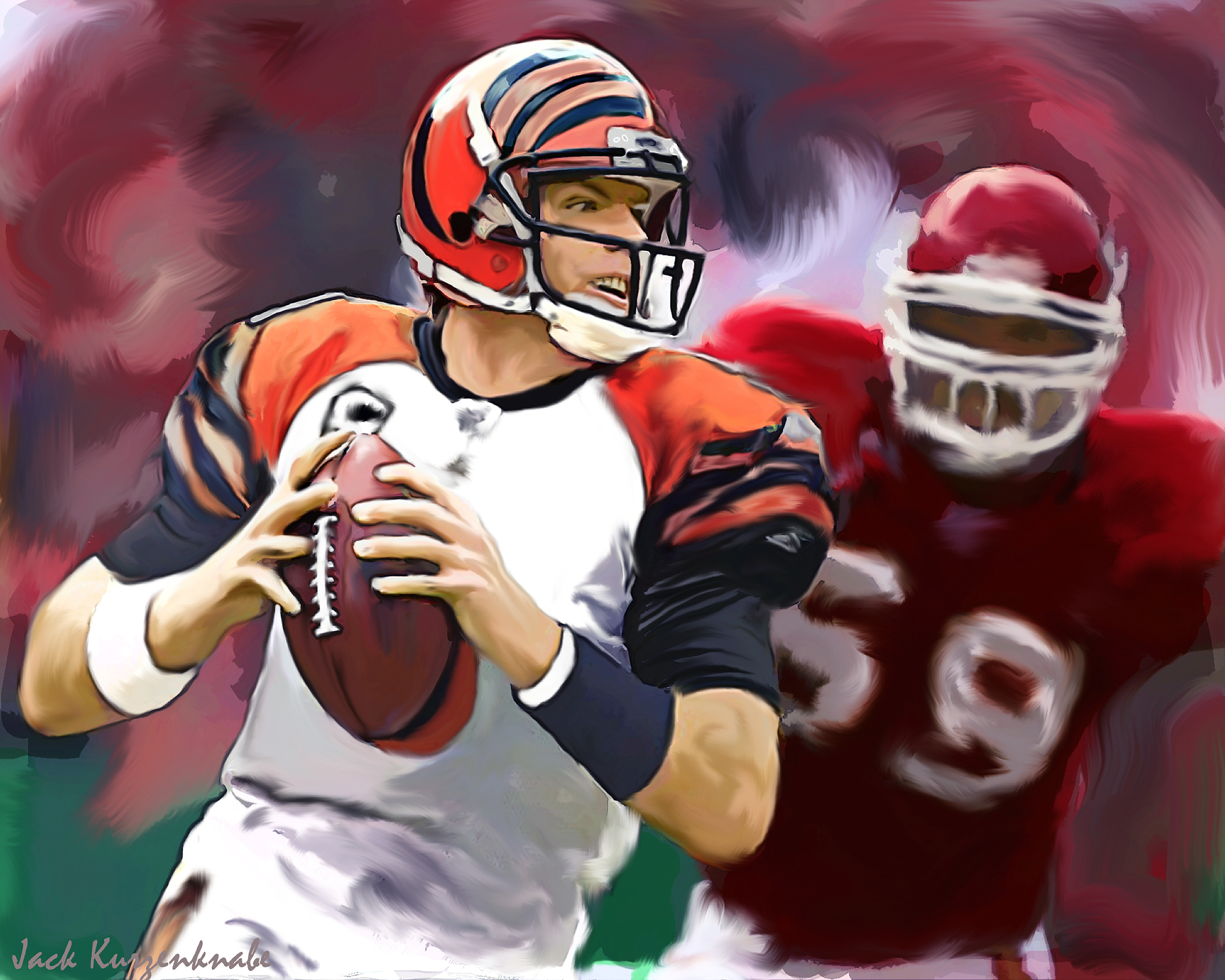This detailed oil painting depicts a dramatic moment in American football. At the center is a quarterback, likely from the Cincinnati Bengals, identifiable by his white jersey with orange and black tiger stripes on the shoulders and his distinctive orange and black helmet with a black face mask. He clutches a red football close to his chest, seemingly poised to throw it downfield. This player also wears a black bracelet on his left wrist and a white one on his right wrist. The chase is on, as a second player in a red jersey with white accents and a red helmet runs close behind him. His jersey is marked with the number 59. The background of the painting swirls with colors of red, white, black, and green, adding a dynamic and artistic flair to the scene. The artist's signature can be seen in the bottom left corner.